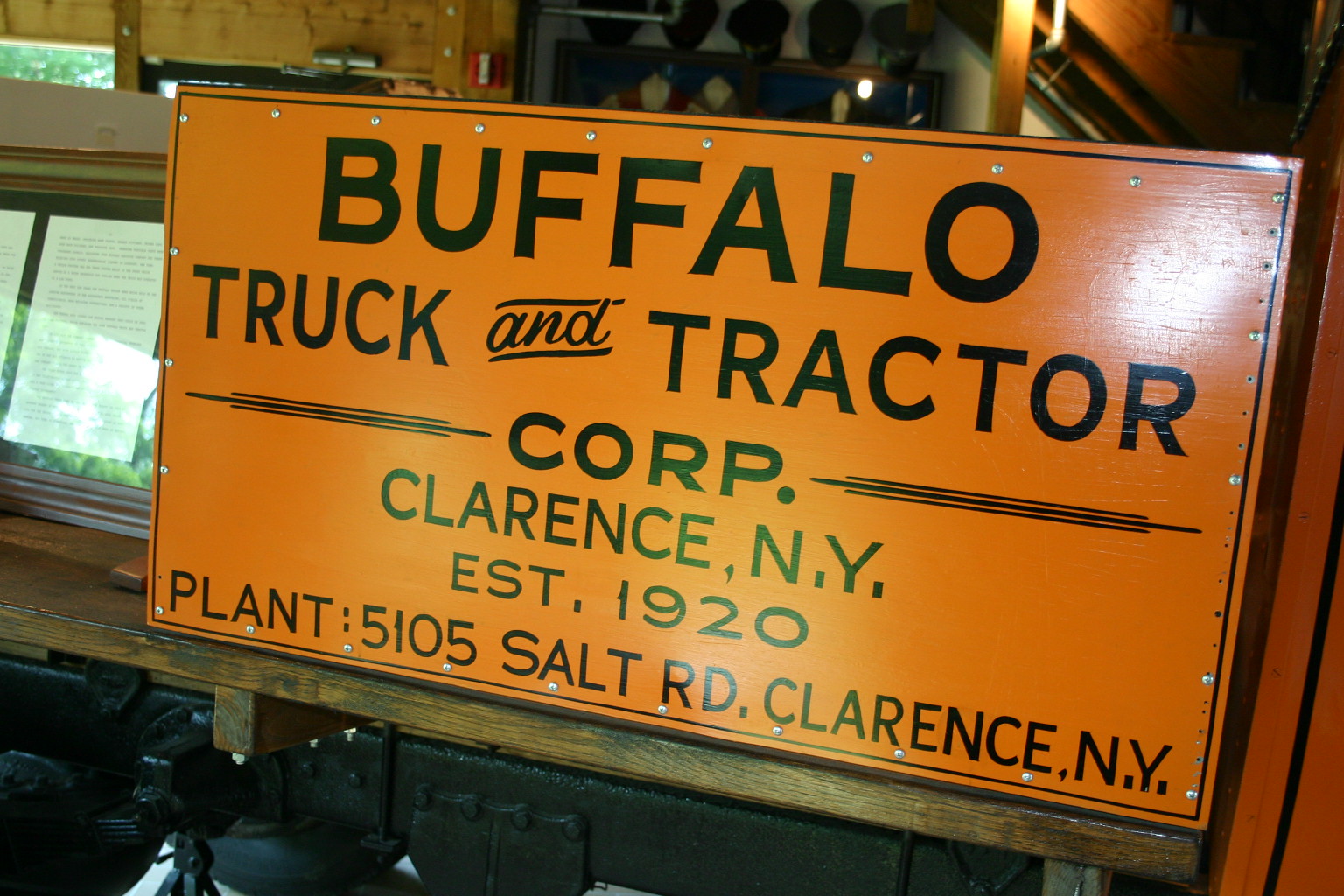This color photograph captures a vintage orange wooden sign with large, neat black lettering, prominently displayed indoors, likely within a museum or workshop setting. The sign reads "Buffalo Truck and Tractor Corp." in large lettering, with "Corp." centered and flanked by three black lines on each side. Below, it states "Clarence, NY, Established 1920," followed by "Plant: 5105 Salt Road, Clarence, NY." The sign is bordered by a thin black line, appearing to be secured with nails or screws. The background features a display case containing 8 1⁄2 by 11-inch papers with writing. A light reflects off the right-hand corner, adding a glint to the scene. Overall, the photo focuses sharply on the sign, making it difficult to discern whether it's attached to a building or part of a window display.